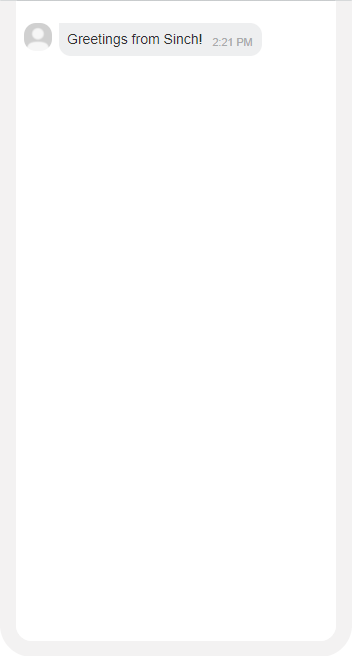The image depicts a mostly blank smartphone screen with grey borders. On the white background, there is a central avatar of a person, accompanied by a message that reads, "Greetings from Cinch!" The message is timestamped at 2:21 PM. The screen itself is predominantly white, surrounded by grey edges, emphasizing the simplicity of the design. The overall visual presentation is minimalistic, with the focus firmly on the greeting message and the avatar.